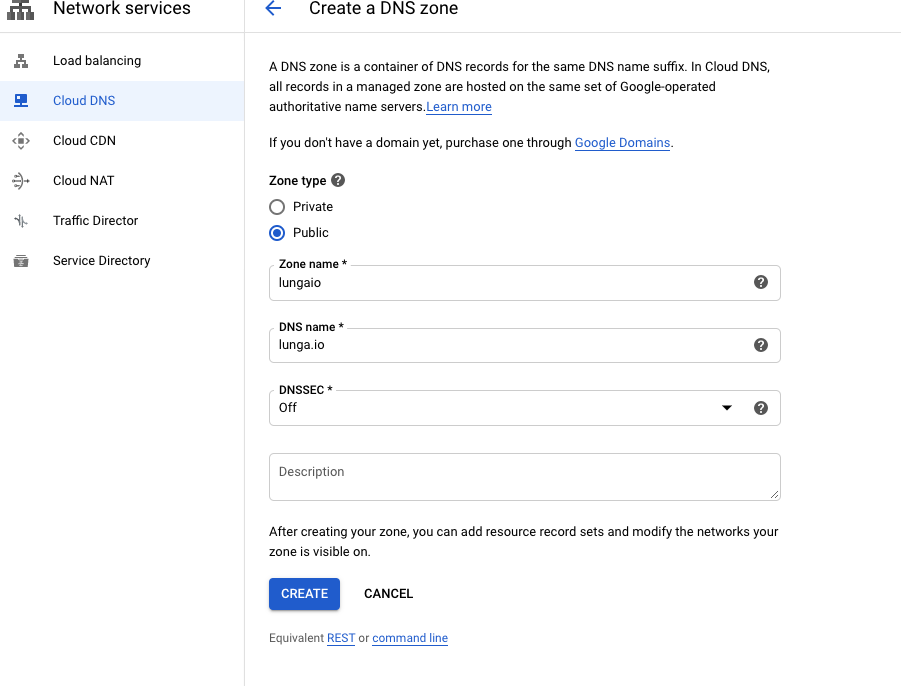This is a detailed screenshot of a computer screen showcasing the Network Services settings, specifically focused on the Cloud DNS tab within the Google Cloud Platform console. 

On the left side, there's a column labeled "Network Services" featuring an icon and several navigational tabs including Load Balancing, Cloud DNS, Cloud CDN, Cloud NAT, Traffic Director, and Service Directory. 

The right side is centered on the Cloud DNS section, identifiable by the highlighted blue tab. At the top, there is a title, "Create a DNS Zone," accompanied by an arrow pointing left, suggesting a back-navigation option. Below the title is a descriptive paragraph explaining that a DNS zone is a container of DNS records sharing the same DNS name suffix. It notes all records within a managed zone are hosted on the same set of Google-operated authoritative name servers. A blue hyperlink titled "Learn more" provides further information on this topic. An additional note mentions, "If you don't have a domain yet, purchase one through Google Domains," also highlighted in blue.

The "Zone Type" section follows, marked by a bold title and a question mark icon for further details. This section offers two selection bullets labeled "Public" and "Private," with the "Public" option currently selected.

Below this, there are four input fields: "Zone Name," "DNS Name," "DNSSEC," and "Description." The first three fields are marked with asterisks to denote mandatory information, each accompanied by a question mark icon for hints or help. These fields have been filled out with data, while the "Description" field remains empty.

At the bottom of the form, an instructional note explains, "After creating your zone, you can add a resource record set and modify the network so your zone is visible." There are two action buttons underneath this message: a blue "Create" button and a black "Cancel" button. The very bottom of the screen offers a link to the "Equivalent REST or command-line" instructions for users preferring alternate methods.

Overall, this screenshot provides a thorough view of the process for creating and configuring a DNS zone within the Google Cloud Platform's Network Services settings.